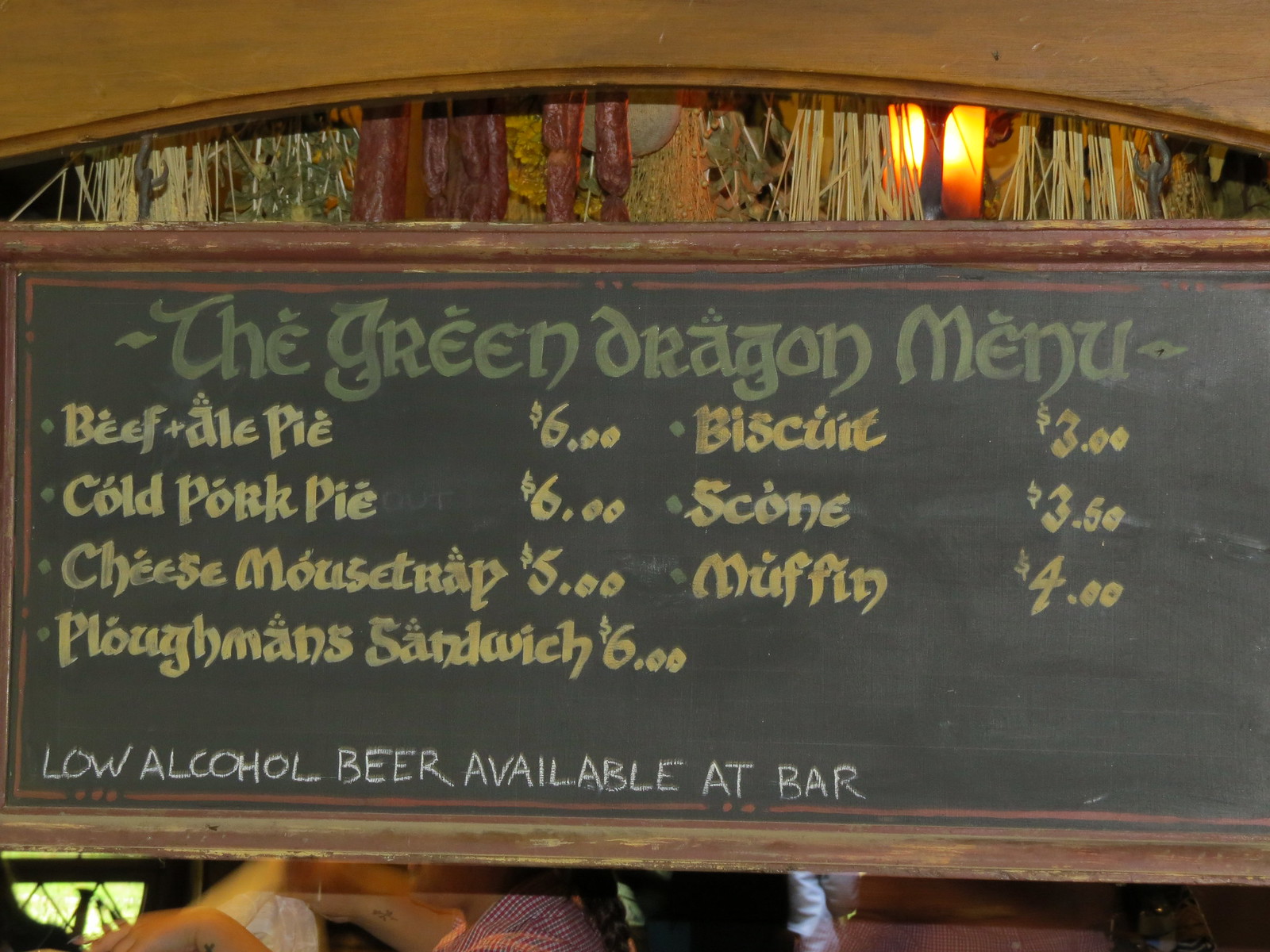This photorealistic image appears to be taken inside a rustic-themed restaurant. The focus of the photograph is a blackboard menu bordered by a dark brown, weathered wooden frame. At the top of the menu, written in ornate, green old-fashioned text, is "The Green Dragon Menu." The menu items are listed in yellow ornate text, featuring: Beef & Ale Pie ($6); Cold Pork Pie ($6); Cheese Mousetrap ($5); and Plowman's Sandwich ($6), all on the left side. On the right side, a separate column lists: Biscuit ($3); Scone ($3.50); and Muffin ($4). Near the bottom left-hand side of the menu, in white text, it reads: "Low alcohol beer available at bar."

Behind the menu, the ceiling features rustic decorations, including dried plants, grasses, and sausages hanging from a wooden beam that runs horizontally across the image. The background also includes some glimpses of lighting and partial views of seated patrons, adding to the warm, authentic ambiance of the venue. The scene exudes a cozy, old-world charm, suggestive of a tavern or countryside inn.